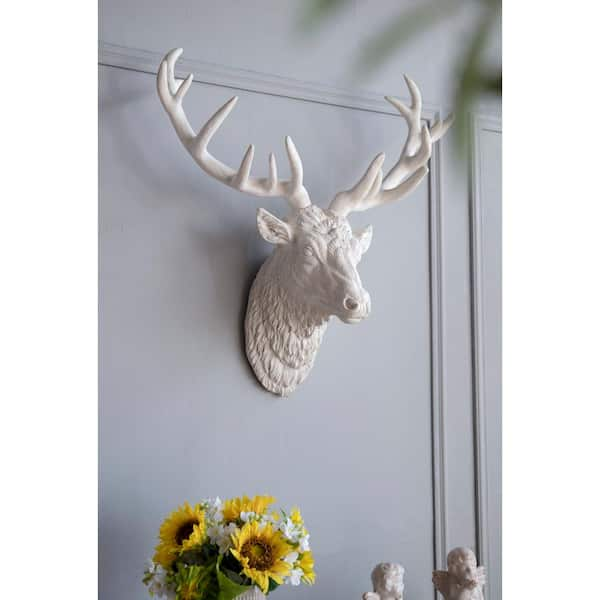The image depicts a detailed sculpture of a deer's head, painted entirely in an ivory white color, mounted on a clean, light gray wall. The sculpture, which may be a taxidermy piece painted white or a replica, showcases intricate details such as the fur, eyes, nostrils, and ears. The deer's head is slightly turned to the right, revealing most features of the left side of the face, with large antlers extending prominently from either side. Each antler has at least six points, though the exact number is difficult to distinguish due to some points being clustered together. Below the deer head, on the bottom left of the image, there is a bouquet of sunflowers and other white flowers. On the bottom right, you can see two baby angel figurines, also painted in a whitish hue. The image is bright and clear, capturing the fine details of the sculpture and the wall it is mounted on.